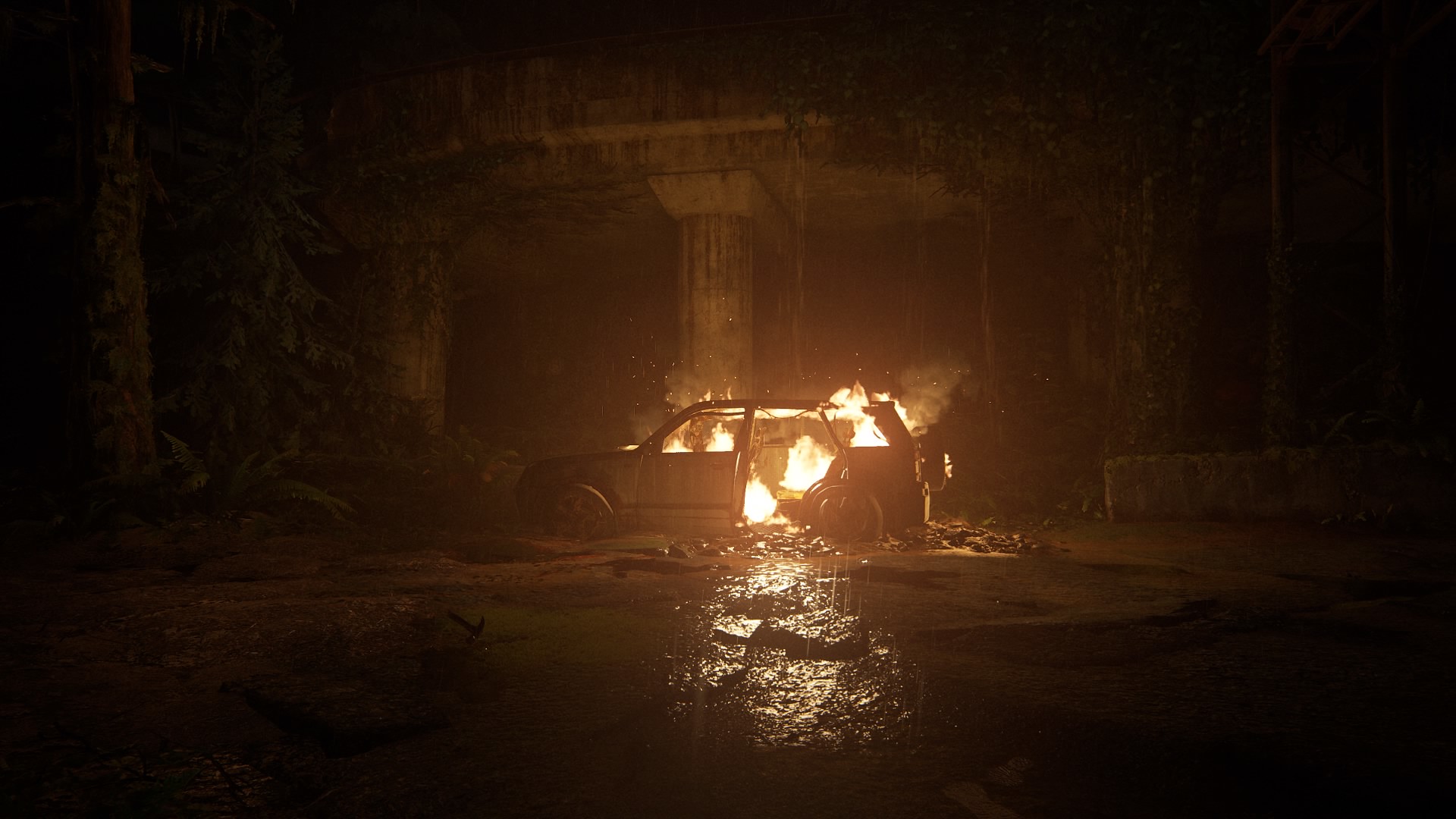This nocturnal image captures the haunting scene of a burning hatchback, set amidst an ambiguous backdrop dominated by darkness and sporadic structures. The primary source of light is the intense blaze from within the car, which starkly highlights the immediate surroundings. The hatchback, significantly damaged and missing its back door, appears engulfed in flames internally, suggesting an explosion or severe impact. The inferno illuminates falling raindrops, which are visible only near the vehicle, adding an eerie shimmer to the chaotic scene. Amidst the vague locale, several large columns, reminiscent of temple ruins or underpass supports, rise in the background. Parts of the car, including door frames and potentially a wheel, are twisted and contorted, further emphasizing the violent nature of the incident. A reflective puddle lies nearby, with scattered pavement and rocks hinting at the crash’s aftermath. The setting's murky details and the mysterious archeological or urban ruin context evoke an ominous and dramatic narrative.